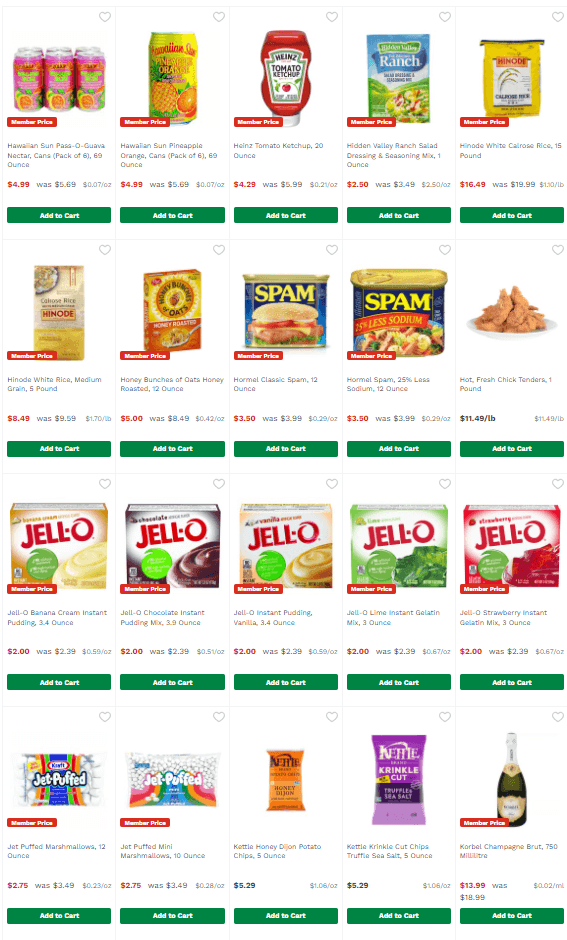This image depicts a detailed section of a grocery website, showcasing a range of items available for purchase. The layout consists of four rows, each with five distinct products, all set against a clean white background. Below each item, a green "Add to Cart" button with white text is prominently displayed. Additionally, a red "Member Price" sticker is visible on most items, indicating special pricing for members.

Starting at the top row, the first item is a six-pack of Hawaiian Sun Pass-O-Guava Nectar cans priced at $5. Next is another Hawaiian canned item, followed by bottles of ketchup, ranch seasoning, and a packet of white rice.

In the second row, the selection continues with another packet of white rice, a box of Honey Bunches of Oats cereal, regular Spam, low-sodium Spam, and hot fresh chicken tenders priced at $11.49 per pound.

The third row features a variety of dessert mixes, including boxes of instant pudding mix and Jell-O gelatin mix.

Finally, the last row includes two bags of marshmallows (one in regular size and the other mini), two bags of kettle-cooked chips, and a bottle of champagne, rounding out the diverse product lineup available on this grocery shopping platform.